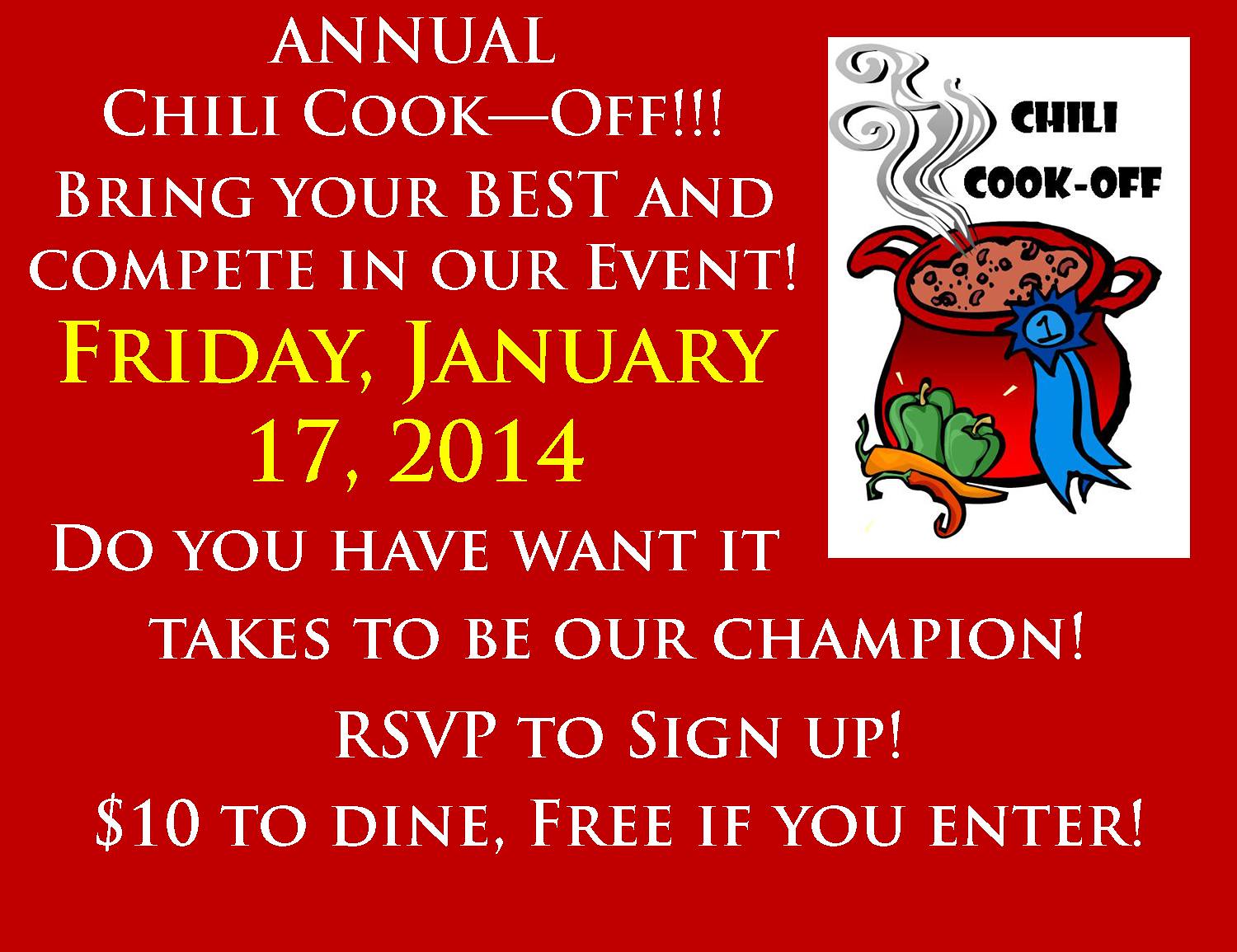The image is a bright red, square-shaped flyer advertising an "Annual Chili Cook-Off!" event. The bold, white capital letters at the top announce "ANNUAL CHILI COOK-OFF!!!" Below it, the text encourages, "Bring your best and compete in our event!" In large, prominent yellow letters, the date "Friday, January 17, 2014," is spotlighted. Further down, in white text, it challenges readers with, "Do you have what it takes to be our champion?" and prompts, "RSVP to sign up." An additional note indicates a cost: "$10 to dine, free if you enter."

On the upper right-hand corner of the flyer, there is a white rectangle featuring a cartoonish image of a chili pot. The pot is red with brown chili inside and white smoke rising from it. A blue ribbon with the number "1" adorns the pot, and surrounding it are green and red peppers. The caption above the image reads "Chili Cook-Off" in black writing.